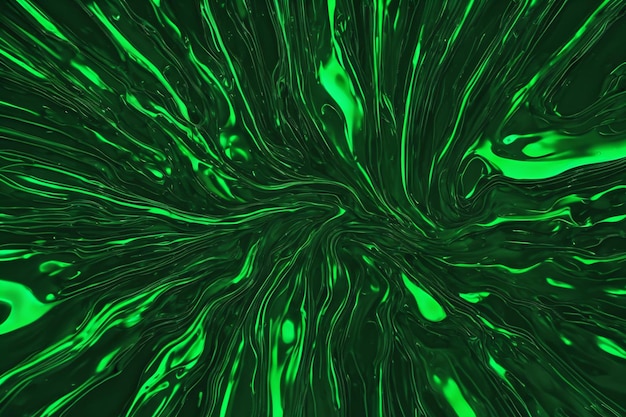The image depicts an intricate swirl of green liquid, possibly a mixture of colored dye, oil, and water, or it may be a digitally crafted composition. The green hues range from dark forest green to almost neon green, with the lighter splotches notably concentrated in the bottom left and top right corners. The liquid appears thick and viscous, giving it an oily consistency. The swirls in the liquid are random yet organically patterned, creating a sense of movement. The symmetry is subtle, with the tops and bottoms flaring out in similar directions, enhancing the wavy, undulating characteristics. The overall effect is akin to viewing a microscopic close-up of a dyed substance with a metallic sheen, or perhaps a computer-generated fluid dynamic simulation, giving an impression both surreal and vividly detailed.